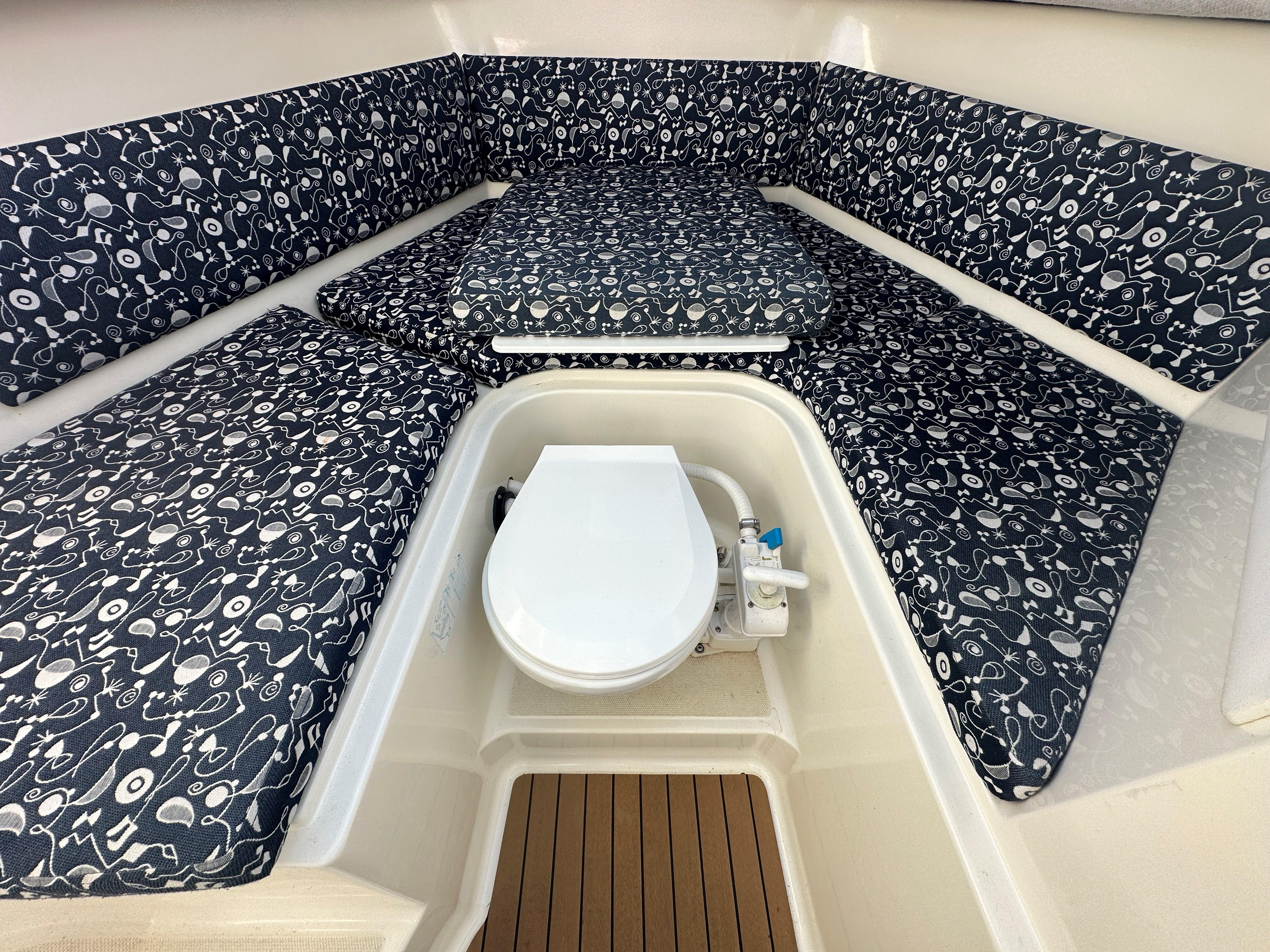The image depicts a section of what appears to be a boat, characterized by surrounding fiberglass walls. At the center of this setup is a toilet with its lid down, possibly a chemical toilet. To the right of the toilet, some mechanisms and tubing are visible, hinting at a bidet or valve system. A noticeable step down in front of the toilet reveals a wooden board or mat. The area around the toilet is cushioned with pads resembling those used in outdoor furniture, stretching across three sides in a triangular shape. These cushions display an abstract black and white design consisting of squiggly lines and symbols. On top of the toilet rests a cover or table in a blue and white pattern, adding to the peculiar juxtaposition of a toilet amid ample cushioned seating. The overall layout and materials suggest a multifunctional, albeit oddly arranged, space within a boat.